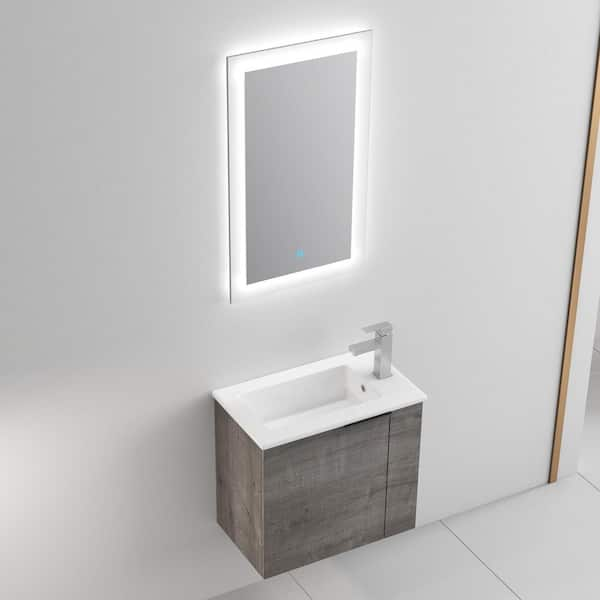The image portrays a sleek and minimalistic bathroom characterized by its modern design and simplicity. Dominating the scene is a large, flat, white wall adorned with two key fixtures. Central to the composition is a floating cabinet made of ashy gray wood, supporting a contemporary rectangular white porcelain vessel sink. Above the sink, positioned slightly to the right, is a brushed nickel faucet. Complementing the sink is a rectangular mirror with a backlit frame that emits a soft glow, enhancing the room's illumination. The setting is further defined by its large square white floor tiles, contributing to the minimalist aesthetic. The overall ambiance is one of modern elegance and understated sophistication.